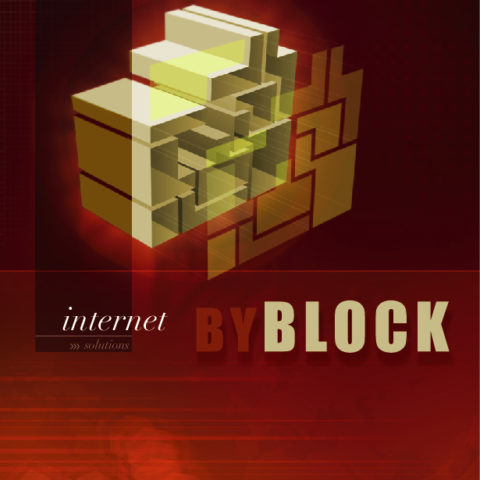The image features a predominantly red background that transitions from darker shades at the top to lighter red shades at the bottom, with a horizontal light red streak cutting through it. At the top of the image, there is a collection of 3D puzzle-like blocks, resembling Tetris pieces in L, T, and square shapes, stacked at various angles. These blocks are superimposed over a 2D design of the same pattern, creating a layered effect. To the left side, a darker red vertical bar contains the text "internet" in white italics above the word "solutions" in smaller, nearly red font. Adjacent to this, in large red capital letters, is the word "BY", followed by the word "BLOCK" in an off-white color. Overall, the caption reads: "Internet solutions by BLOCK."